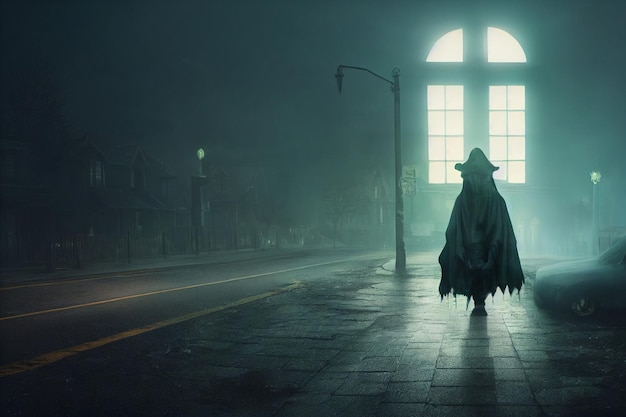The image portrays a hazy, night-time outdoor scene featuring a single cloaked humanoid figure standing on a worn, cobblestone pedestrian walkway that blends into a black asphalt road marked with yellow and white lines. To the right of the figure is a car, seemingly missing its tires and covered in a layer of mist or dust. The figure, who appears tall with a pointed tricorn hat and a thick white cloak draping down to their feet, stands to the right of a street light. They are silhouetted against a large, floating windowpane that emits a bright light, illuminating the surrounding area, including the car. The glowing window, positioned in the back right of the scene, appears mysteriously detached from any building, thereby creating an ethereal, almost dreamlike atmosphere. In the distance, other houses can be barely discerned, adding to the surreal quality of the image.